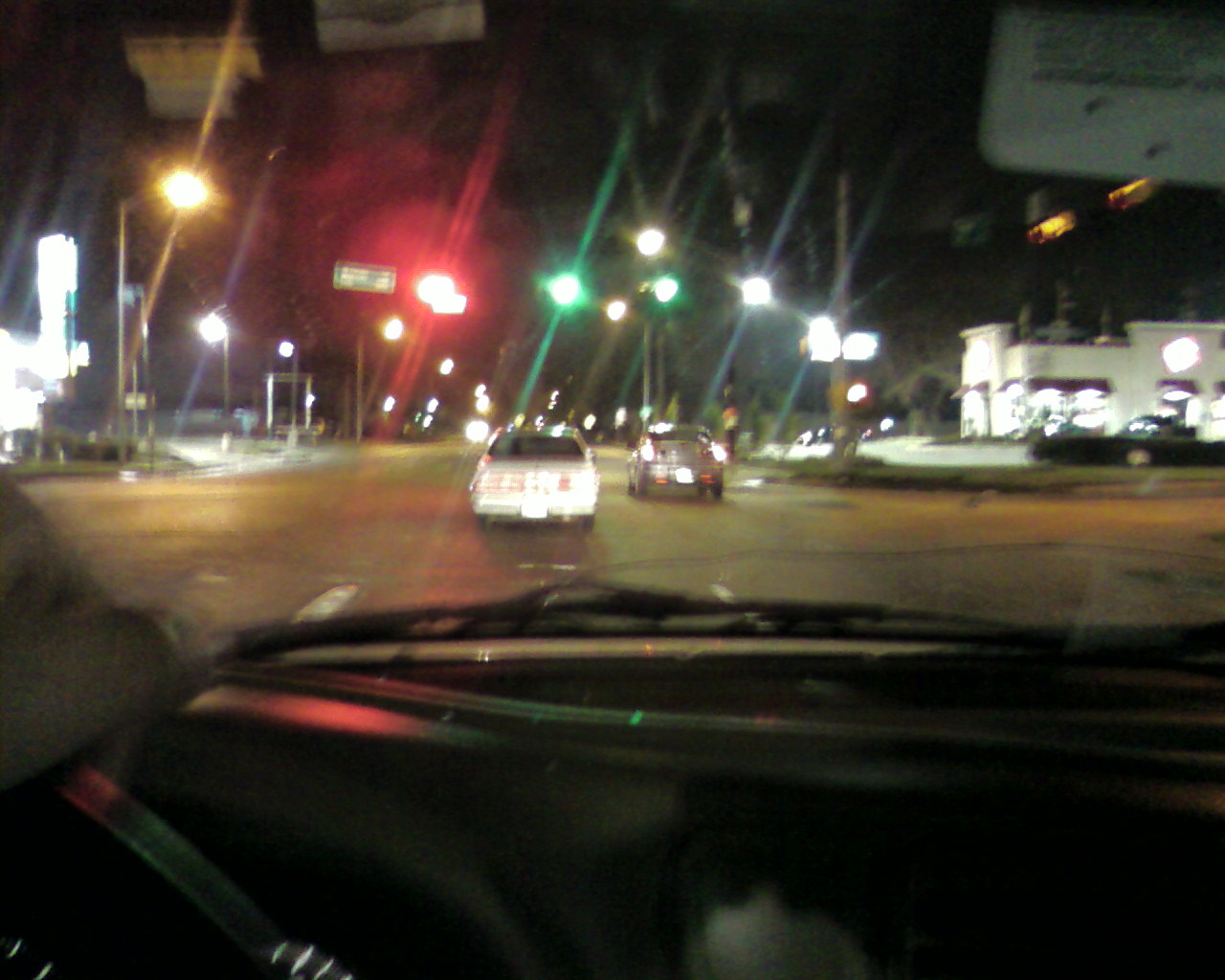This nighttime photograph is taken from inside a car, through the front windshield. The sky is an inky black, setting a stark contrast for the scene ahead. Inside the car, parts of the dashboard and windshield wipers are just visible. The road stretches out in front with a few vehicles on it. A white car is directly ahead, while a grayish-brown car is slightly to its right. The street is adorned with a variety of lights—green, red, white, and a solitary yellow light on the left side of the road. On the right side, there appears to be a one-story restaurant, warmly lit from within, showcasing numerous windows. Additional structures populate the right side, though they are less distinct. The overall ambiance is a mix of illuminated urban life against the tranquil darkness of the night.